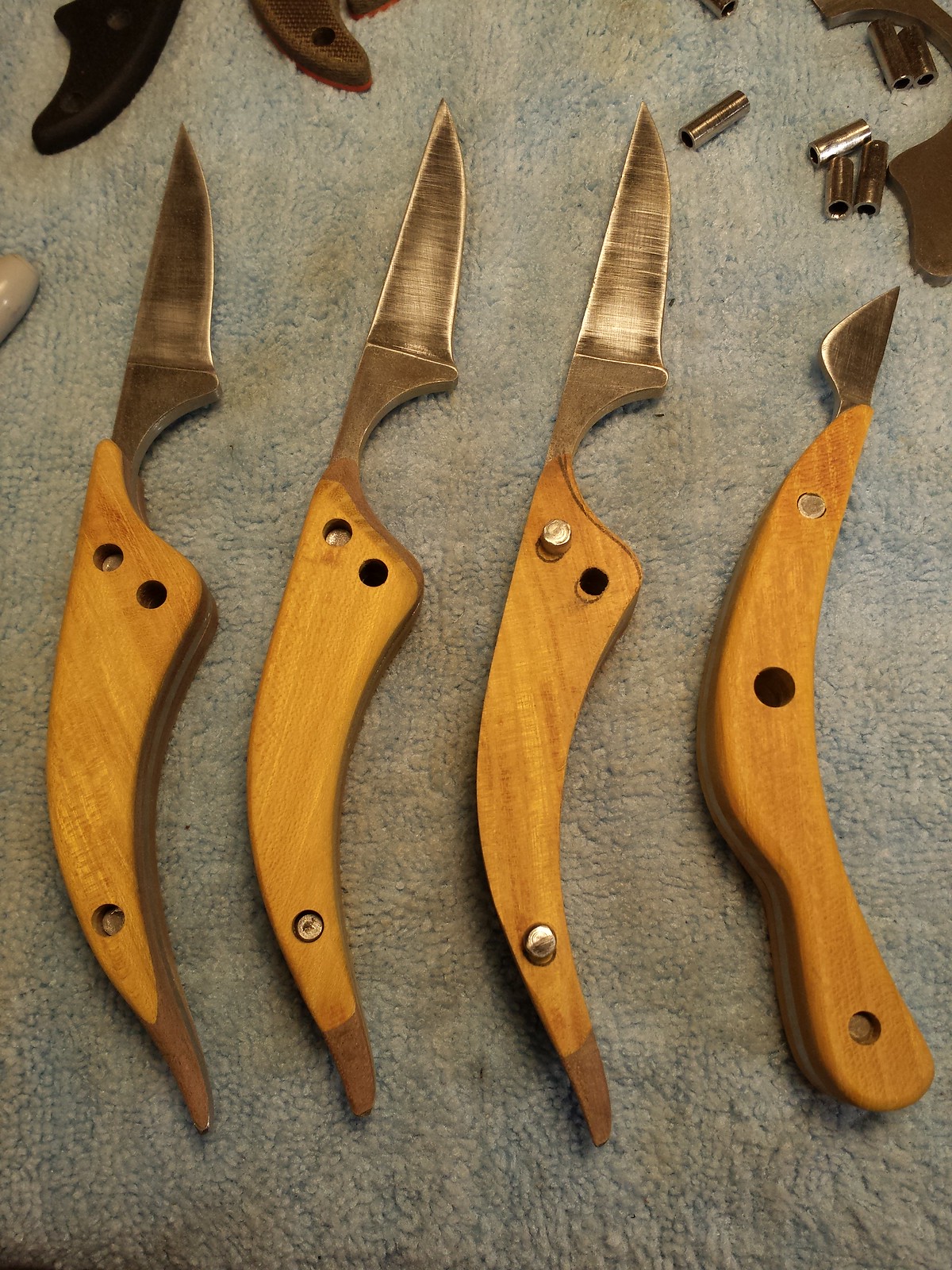In the image, a series of four antique-looking pocket knives are meticulously lined up from left to right on a tan, leather-like surface. Each knife features a handle crafted from a light maple-colored wood, with a slight curve for ergonomic grip, secured by three rivets. The blades, although short, are triangular and dark silver with markings indicative of sharpening. Notably, the base of each blade forms an arched area where the handle meets the blade, allowing for finger stabilization. In the upper right corner of the photograph are loose, hollow metal cylinders, and in the upper left corner, there are fragments of brown leather. The overall arrangement suggests a state of assembly or repair, adding to the intricate historical charm of these pocket knives.